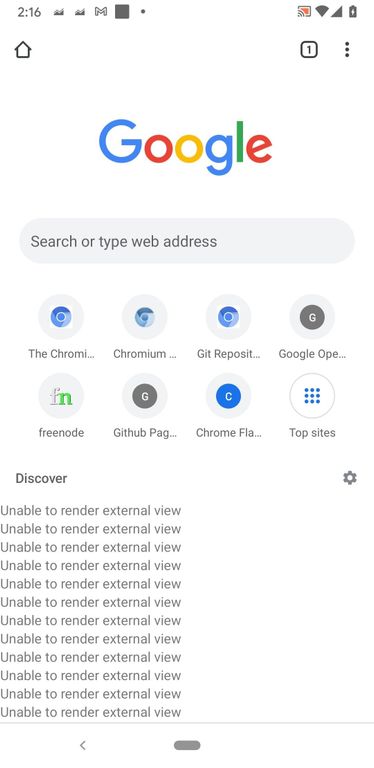The image is a screenshot of a Google site displayed on a device, possibly a phone or tablet. At the top, there is a small house icon, along with the time (2:16) and several other icons on both the left and right sides. On the right side, there is also a camera icon and a battery indicator showing the device's power level.

Centered prominently in the image is the Google logo, featuring the well-known multicolored letters: a big "G" and a small "g" in blue, the first "o" and the "e" in red, the middle "o" in yellow, and the "l" in green. Below this logo, there is a search bar with the prompt "Search or type web address."

Under the search bar, there are eight icons arranged in a grid. Some of these icons are partially cut off, represented by ellipses (...). Most of the icons resemble the circular Google design, which typically features a dot in the center (colored blue in this case) surrounded by a slightly larger blue circle, with space between the two circles.

The specific icons and their labels are:
1. Chromie
2. Chromium
3. Git Reposit
4. Google OPE
5. Free Node (with an "fn" in the icon)
6. GitHub Pag (with a "g" in the icon)
7. Chrome Fla (with a "c" in the center of the blue circle)
8. Nine dots labeled as "Top sites"

Below these icons, there is a repeated message in gray text: "Unable to render external view," appearing eight times in a row, each line stacked on top of the other.